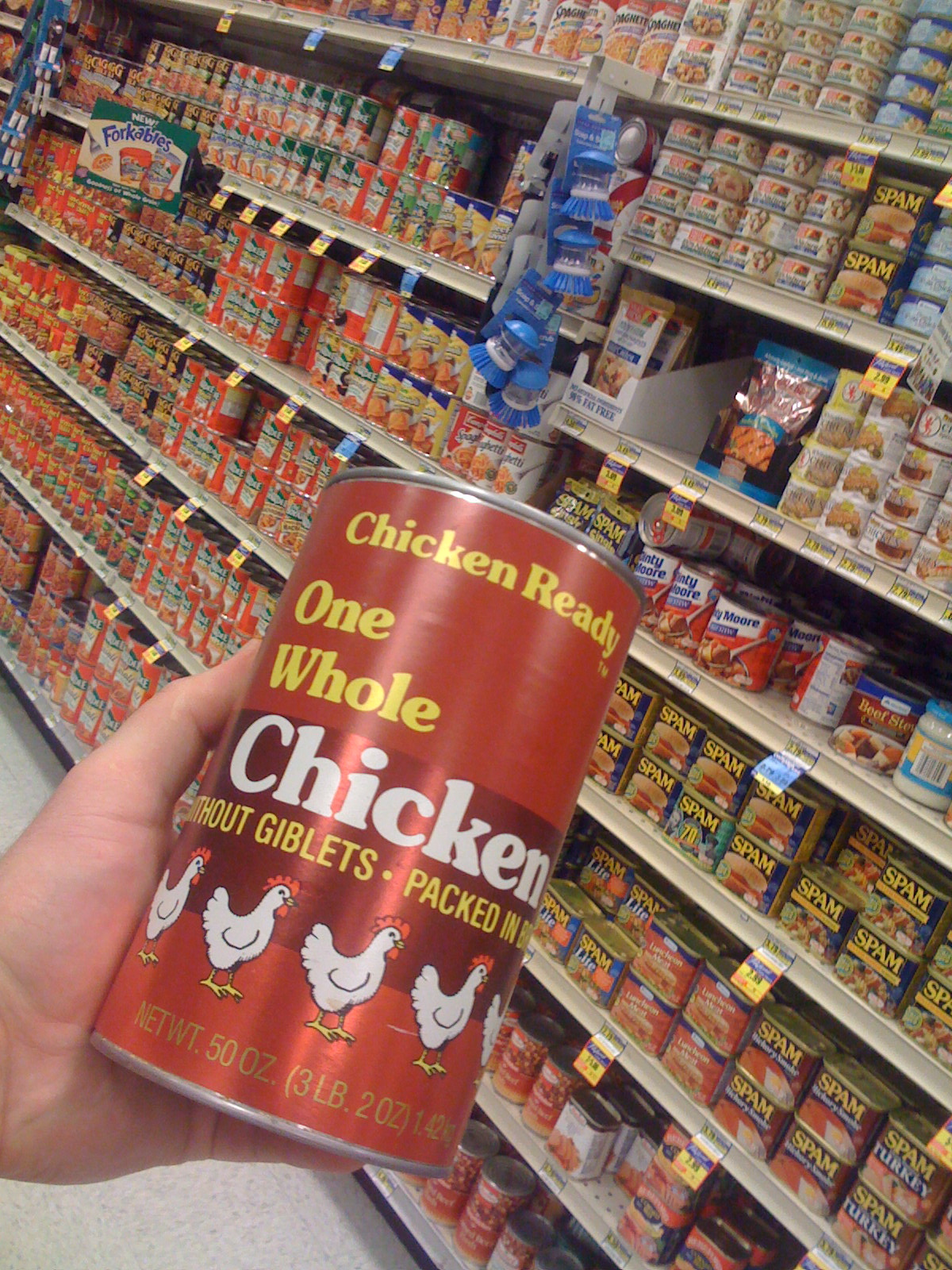In this photograph, a person with a fair-skinned hand is holding a can labeled "Chicken Ready" in the center. The can is prominently red with bold yellow lettering at the top, stating "Chicken Ready" followed by white lettering that reads "One Whole Chicken with Giblets." The can, which is likely made of aluminum, displays several small illustrations of chickens in various poses below the text, each depicted in white and red with yellow feet.

The background reveals a shelving unit stocked with similar cans, prominently featuring red labeling. Other items, like blue-labeled Spam cans, are noticeable in the lower right corner. The setting appears to be a grocery store, with neatly lined rows of canned goods displayed on metal shelves. The floor is composed of white tiles, adding to the typical appearance of a commercial retail environment.